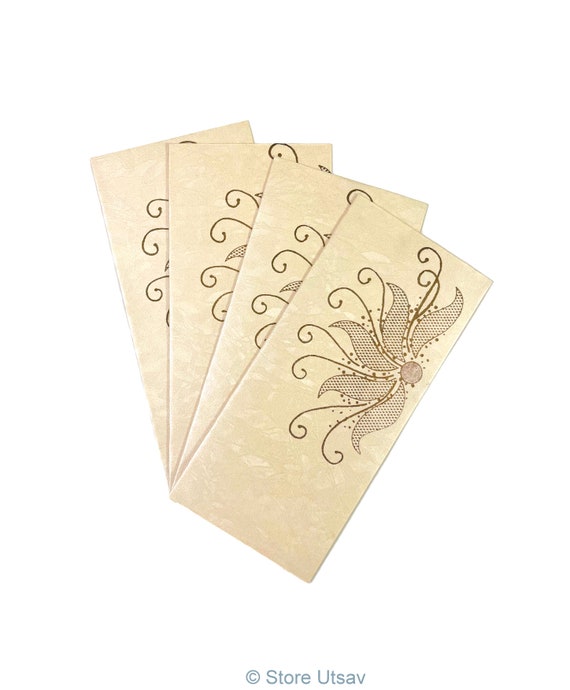This image is a product listing for a pack of four pieces of paper-like items, possibly day planners, budget planners, place cards, or even envelopes. The items are crafted from a yellowish, textured, and slightly stained cardstock that carries a sophisticated, vintage appeal. Each piece showcases a delicate, floral-inspired design made up of intricate dots and lines, forming abstract flower shapes and tendrils. These designs are in brown and gold, giving a rich contrast to the paper's background, which seems to have a subtle pinkish hue. The cards are fanned out in the image, revealing only the complete design on the top card, while the others peep out partially. Notably, the detailed decoration features pointed, leaf-like shapes reminiscent of poinsettia leaves, intermingled with swirling tendrils. At the bottom of each piece, the phrase "copyright store UTSAV" is printed, solidifying their unique and artistic origin.